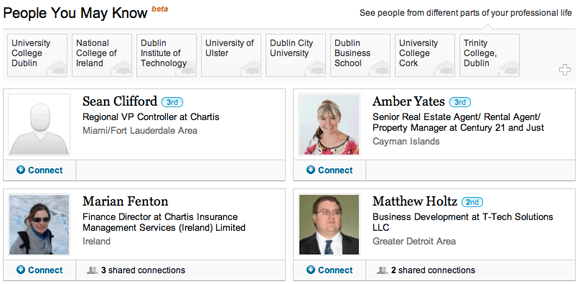Here's a cleaned-up and detailed descriptive caption for the image:

---

The screenshot displays a section titled "People You May Know, Beta" in the top-left corner, with a prompt to "See people from different parts of your professional life" to the right. Below this heading are several tabs, each enclosed in square boxes, listing various educational institutions: University College Dublin, National College of Ireland, Dublin Institute of Technology, University of Ulster, Dublin City University, Dublin Business School, University College Cork, and Trinity College Dublin. To the right of these institutions is a white plus sign, indicating the option to add more colleges for a user searching for former colleagues.

Below this, the profile of Sean Clifford is displayed, identified as a third-degree connection by a blue icon labeled "3rd". He is the Regional VP Controller at Chartis, based in the Miami-Fort Lauderdale area. His profile picture is blank, and there is an option to connect with him via a blue button with a circular plus sign on the left.

Further down, another profile appears for Marian Fenton, the Finance Director at Chartis Insurance Management Services Ireland Limited, based in Ireland. Similar to Sean's profile, there's a blue connect button beneath her blank profile picture. The profile also notes that there are three shared connections to her right.